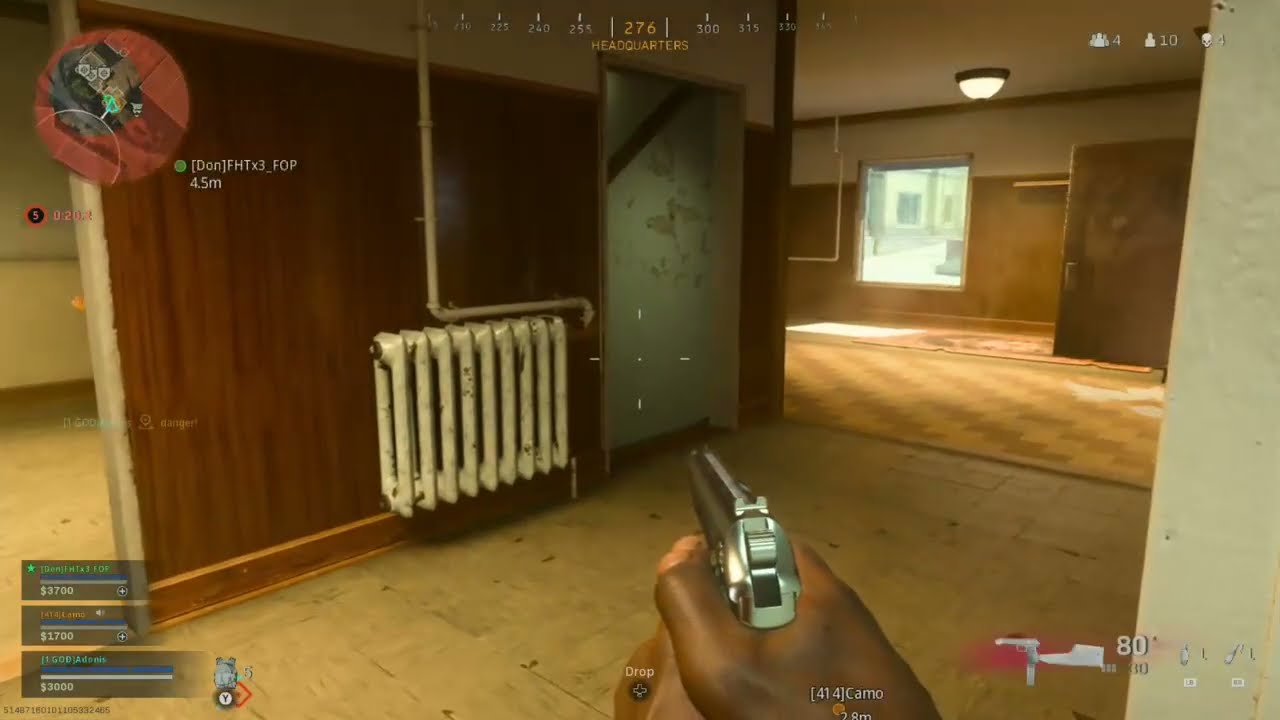The image is a highly detailed, color screenshot from a first-person shooter video game. It features an African American character's hands holding a silver pistol in a two-handed grip, centered in the foreground. The scene is set inside an old, possibly abandoned building with predominantly brown hues and wooden panel walls. The floor transitions between tile and wood. 

To the right of the main room, an entryway leads into another room with a checkered floor and a single visible light. A white, old-fashioned radiator, indicative of older apartment heating systems, is mounted on the wall facing the player. A window in the adjacent room suggests daytime, showcasing an outside building. 

In-game statistics and icons are visible at all four corners of the screen: a circular map with red symbols occupies the top left, additional stats are present on the bottom left, and more indicators fill the top right and bottom right corners. This immersive setting is indicative of a shooting-based video game environment.